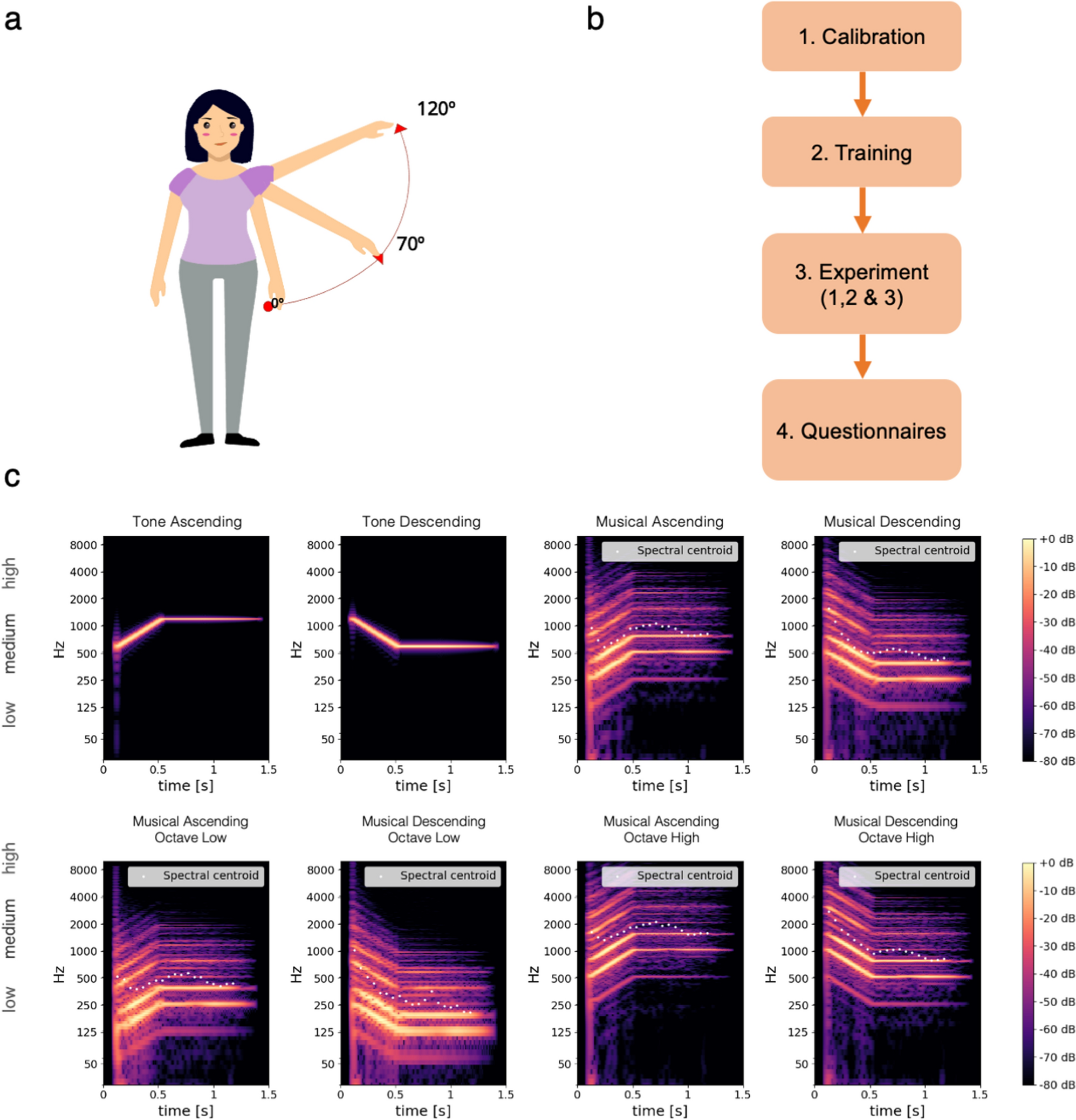The diagram is divided into three sections: A, B, and C. In Section A, there is a cartoon woman with short black hair wearing a purple top and green pants. She demonstrates arm movements by raising her left arm at 0 degrees, 70 degrees, and 120 degrees. Section B lists four items: collaboration, training, experiment 1, 2, and 3, and questionnaires. In Section C, there are eight graphs on a black background with purple and pink lines. The graphs illustrate various musical notes and tones, showing data for tone ascending, tone descending, musical ascending, musical descending, musical ascending octave low, and musical ascending octave high. Each graph is labeled with corresponding numbers on the sides.